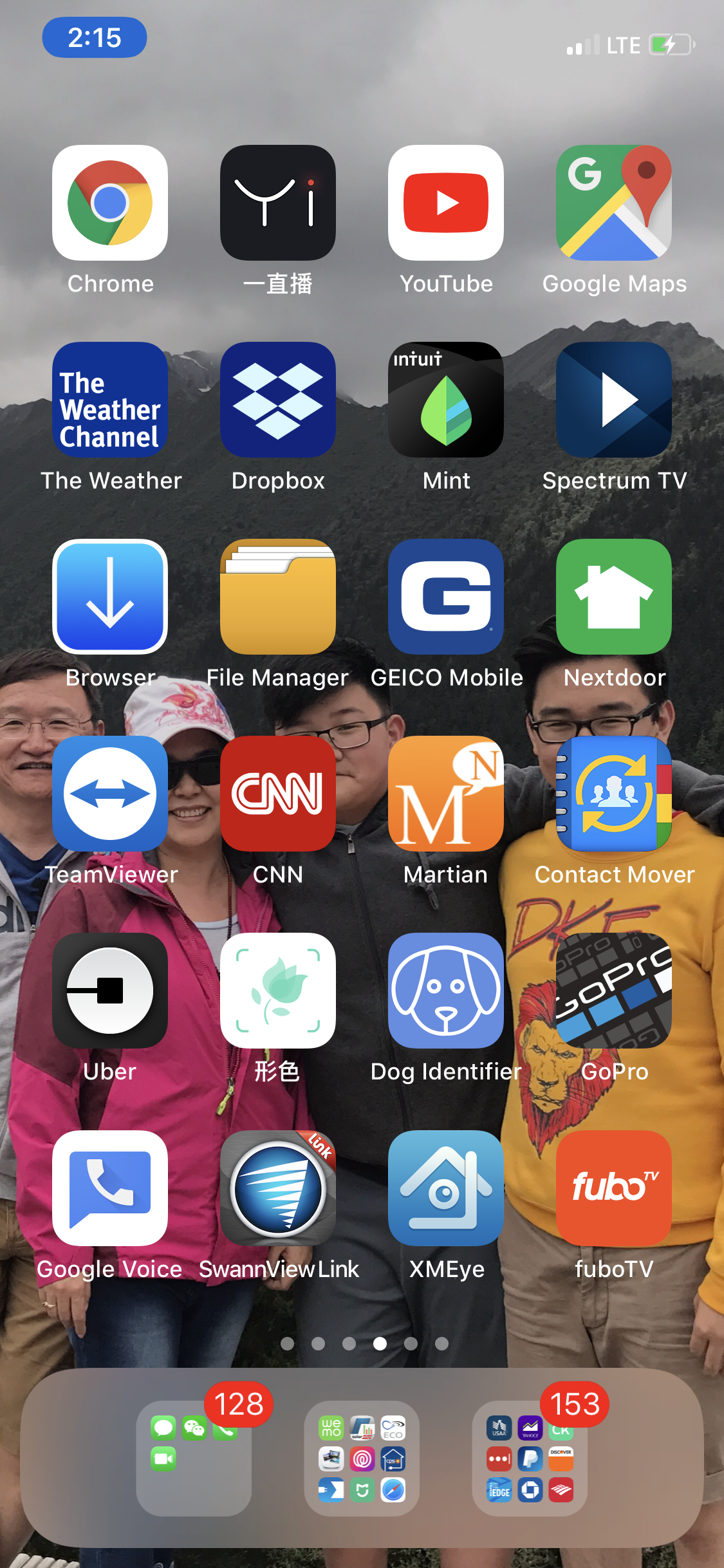This image depicts the home screen of an iPhone, identifiable by its distinctive applications and user interface. The background wallpaper features a family portrait of four Asian individuals set against a backdrop of dark gray, cloudy skies and distant mountains. 

The eldest male in the image wears black-rimmed glasses, has black hair, and is dressed in a white hoodie with black writing, layered over a blue shirt. Standing next to him is an older woman, adorned with black shades and a white and pink hat. She sports a black and pink jacket, a white shirt, blue jeans, and a wedding ring on her left hand.

Beside the woman are two younger males. One wears a black jacket, gray shorts, black glasses, and has black hair. The other is dressed in tan shorts and a yellow shirt decorated with a red tiger or lion, also sporting black glasses and black hair.

The phone's status bar shows an LTE signal and a time of 2:15. The home screen displays a multitude of applications, and notably, there are numerous notifications: 128 in one section and 153 in another.